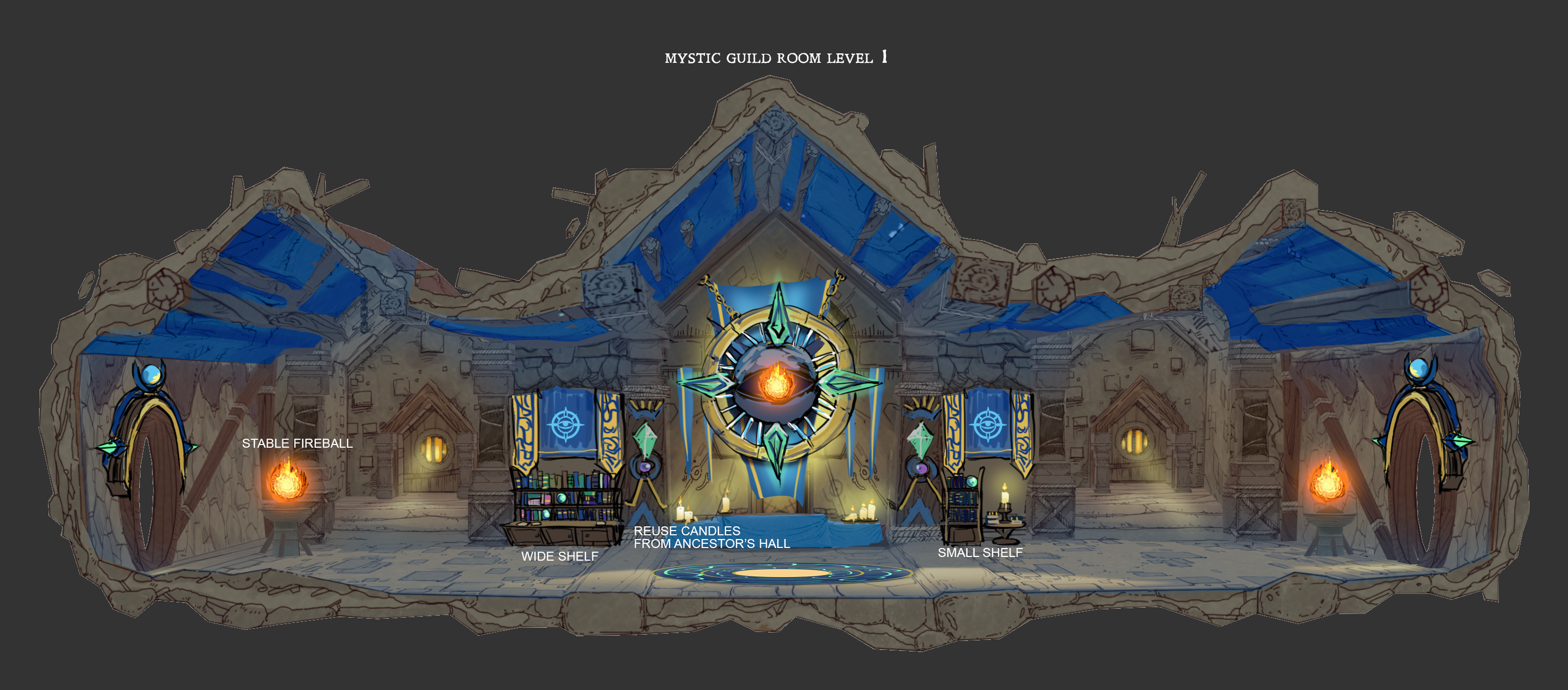This image is a detailed computer graphic taken from a fantasy video game, possibly resembling World of Warcraft or Dungeons and Dragons. Titled "Mystic Guild Room Level 1," it showcases a wide shot of what appears to be an ancient guild room inside a cave. The room is predominantly brown, constructed from rock and wood, with the ceiling giving off a bluish glow, likely illuminated by ambient magic lights.

In the center of the room is a large, fiery altar, featuring a burning red fire encased within a circle and flanked by four green crystals — one positioned to the north, south, east, and west. Surrounding the altar, there are candles, crystals, and side banners, all further contributing to the mystical atmosphere. Text labels within the room highlight various objects, such as a "Wide Shelf" and a "Small Shelf". Another text prompt, "Reuse Candles from Ancestors Hall," suggests an interactive or instructional element within the game.

The space is lit by flames, giving it a magical ambiance with red flames casting a glow onto the surroundings. There are also two prominent doorways — one on the far right and one on the far left, likely serving as entrances or exits for the player. The overall scene combines medieval architectural elements with mystical or magical aesthetics, including rounded doors and crystalline features.